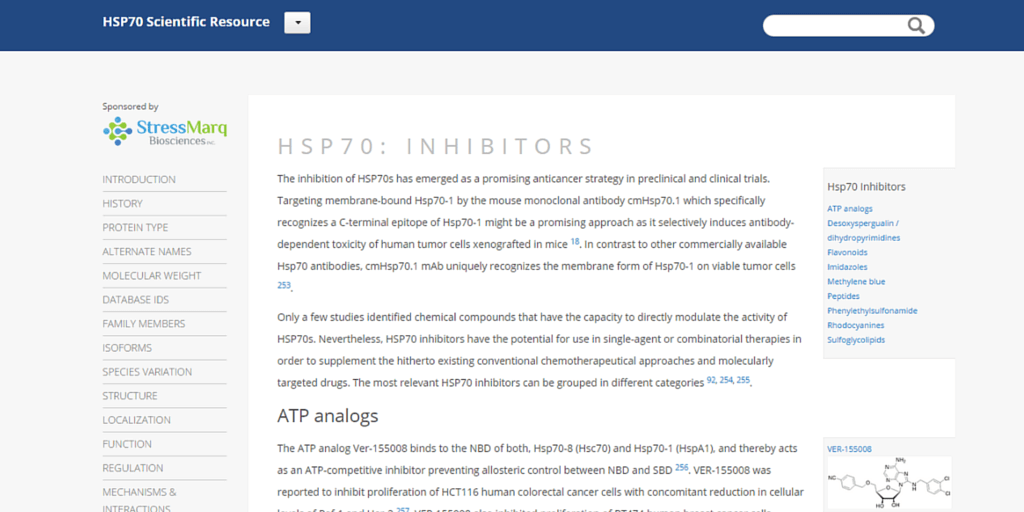The image is a screenshot of a research paper titled "HSP 70 Scientific Resource." At the top left corner, the title is prominently displayed. Below the title is a white dropdown box featuring a small downward arrow. On the top right, there is a search bar with a search icon at its end. Dominating the center of the page is the text "HSP 70 Inhibitors," indicating the topic of discussion.

The paper appears to provide a comprehensive overview of HSP 70 proteins, detailing their functions, introduction, and historical context. A subsection titled "ATP Analogs" is visible, suggesting a detailed exploration of these compounds. On the left margin of the page, it is noted that the content is sponsored by Stress Mark Biosciences.

The document is divided into several sections, including "Introduction," "History," "Protein Type," "Alternate Aims," "Molecular Weight," "Database," "Family Members," and "Isoforms," indicating a thorough and structured breakdown of HSP 70-related information.